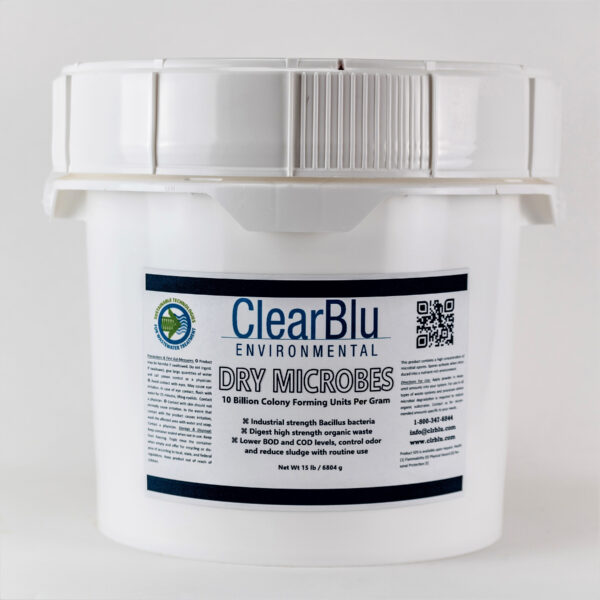This photograph captures a white, plastic industrial bucket prominently displayed against a pure white, square backdrop. The bucket, which has a lid featuring numerous grooves and divots, suggests it is designed to be challenging to open, likely due to its hazardous contents. The bucket is labeled with a white sticker adorned with black bars at the top and bottom. The label features blue and black text, starting with the company's name, "ClearBlu Environmental." Central text reads "Dry Microbes, 10 billion colony-forming units per gram," indicating the contents are industrial-strength bacillus bacteria. Below this, in smaller black letters, the label elaborates: "Digest high strength organic waste, lower BOD and COD levels, control odor and reduce sludge with routine use." At the top right of the label is a QR code, and the bottom includes an 800-number, email address, and website for the company. The top left of the label displays a round blue and green logo with a green arrow and blue waves, accompanied by small writing. The bucket is marked with a net weight of 15 pounds.